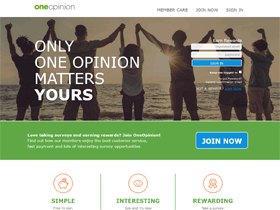The image is a detailed screenshot of the homepage of the "One Opinion" website. The header, which has a white background, features the organization's name styled as "oneopinion," with "one" in green and "opinion" in gray, all in lowercase letters. To the right of the logo, the header includes navigation options: "Member Care" to the far right, "Join Now" to its left, and "Sign In" further to the left.

Below the header is a large, full-width banner image depicting a group of people standing with their backs to the camera, facing a vast body of water. This body of water, extending from one side of the webpage to the other, could be a lake, river, or ocean. The individuals in the image are holding hands and raising them upwards. On the left, there is a woman, followed by a man, a much shorter woman or child in the middle, another man, another woman, and finally a man on the right. The image has a sepia tone, giving it an artistic, timeless appearance.

Overlaying this banner image, a bold white headline in all caps reads, "ONLY ONE OPINION MATTERS, YOURS." The word "YOURS" is emphasized in bold font. To the right of this headline, there is a sign-in form consisting of two white rectangular input fields and a blue rectangular button for submission. Below the sign-in section, there is a green-bordered area with a blue "Join Now" button featuring white capital letters.

Further down, the section's white background showcases the phrases "Simple," "Interesting," and "Rewarding" written in green font, each spaced out and accompanied by a red outlined circle with a small icon above each word.